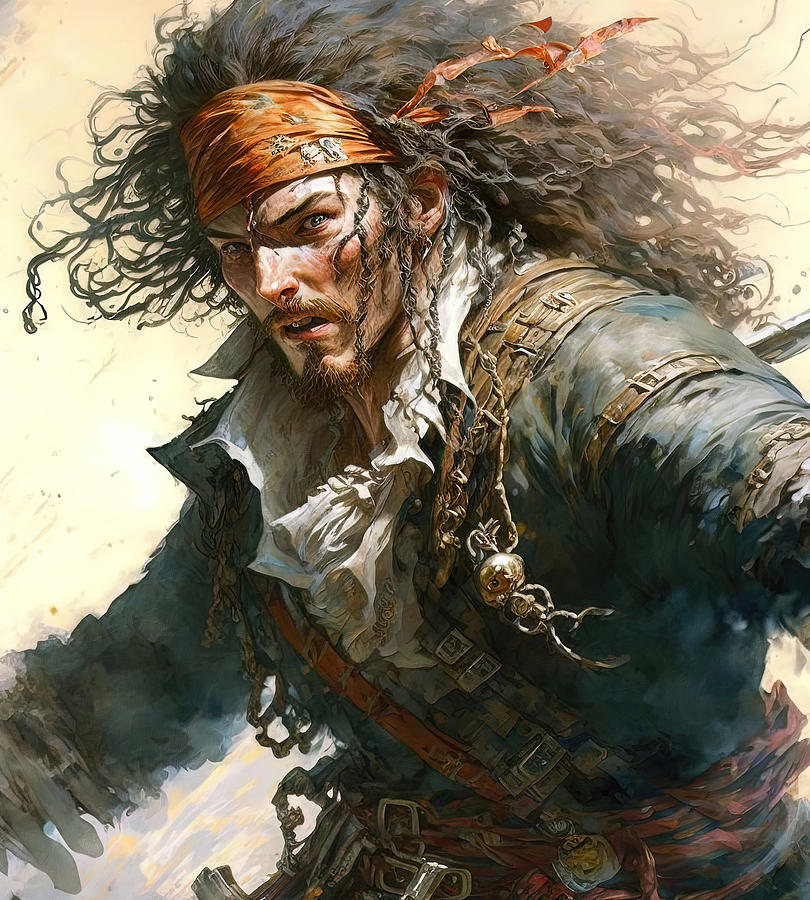This image appears to be a detailed painting or animated poster of a pirate resembling Jack Sparrow from "Pirates of the Caribbean." The pirate stands against a tannish background, dressed in a white ruffled button-up shirt under a blue coat. He is adorned with numerous leather straps and buckles across his shoulders, arms, and chest. His long, curly dark brown hair transitions to a lighter brown at the ends, cascading down behind him. Tied around his forehead is an orange bandana, tattered and decorated with silver pins. His face, sporting a mustache and goatee, bears an expression that seems both angry and fearful as he gazes toward the viewer. He is also equipped with a red rope belt featuring several buckles, adding to his rugged and gritty appearance. His left arm extends off the image, creating a blurry effect in the lower left corner, while his head is positioned at the top left. His uniform also has gold bands on the shoulders and arms, enhancing his pirate ensemble with a touch of detail.